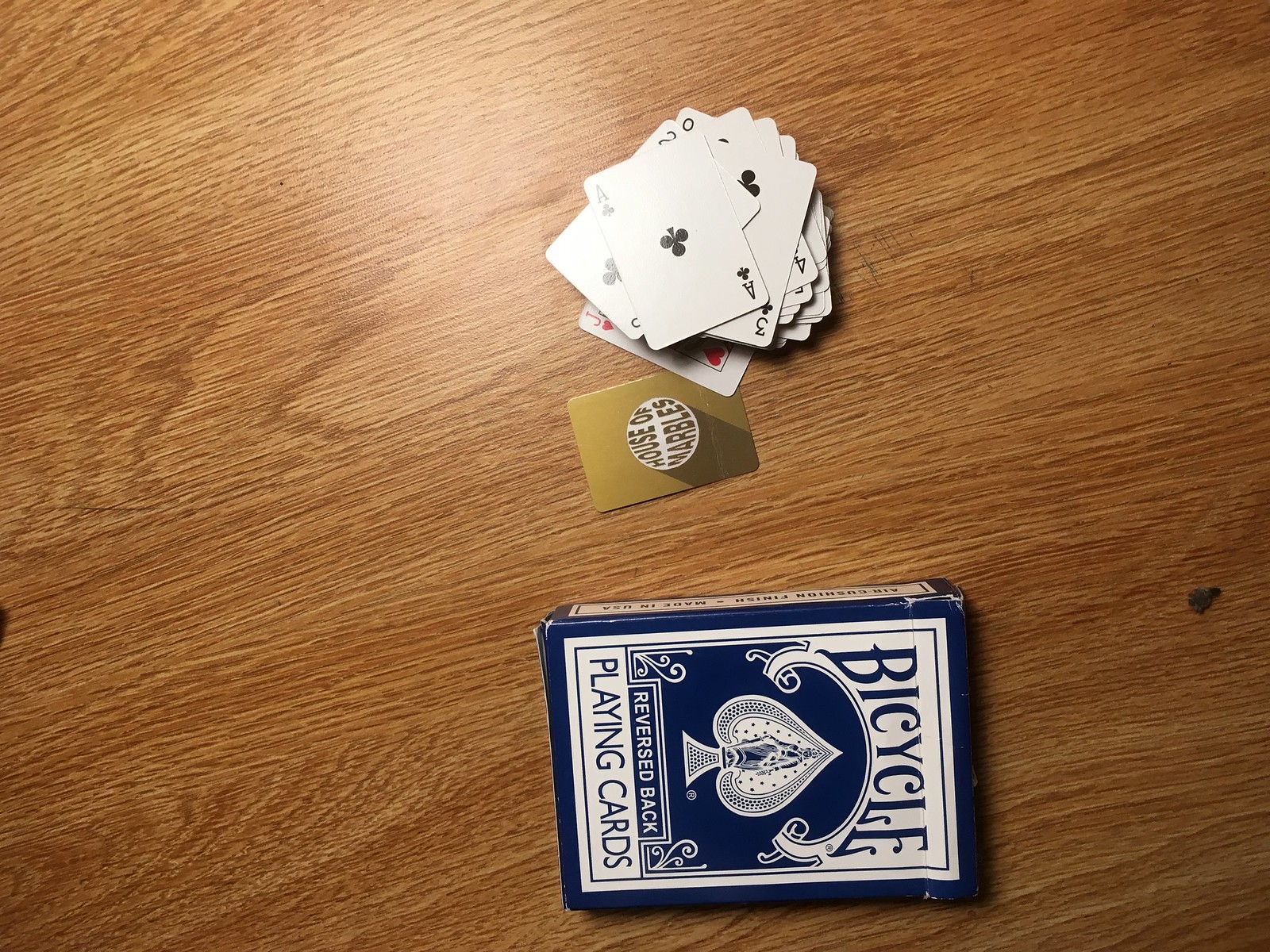The photograph, taken from an aerial perspective, captures a wooden surface covered with a scattered deck of cards. The deck, along with its packaging, is spread out haphazardly. The prominent card on top of the pile is the Ace of Clubs, with the Two of Clubs slightly visible beneath it, followed by the Three of Clubs partially peeking through. Below the Three of Clubs, only the black number four in the corner is visible, leaving its suit indeterminate. Among the disordered pile, the Jack of Hearts can be seen at the bottom edge. A distinct, small gold card marked "House of Marbles" in a white circle is also positioned slightly below the Jack of Hearts. Completing the scene is the empty blue and white “Bicycle Reverse Back Playing Cards” box, lying near the card pile.